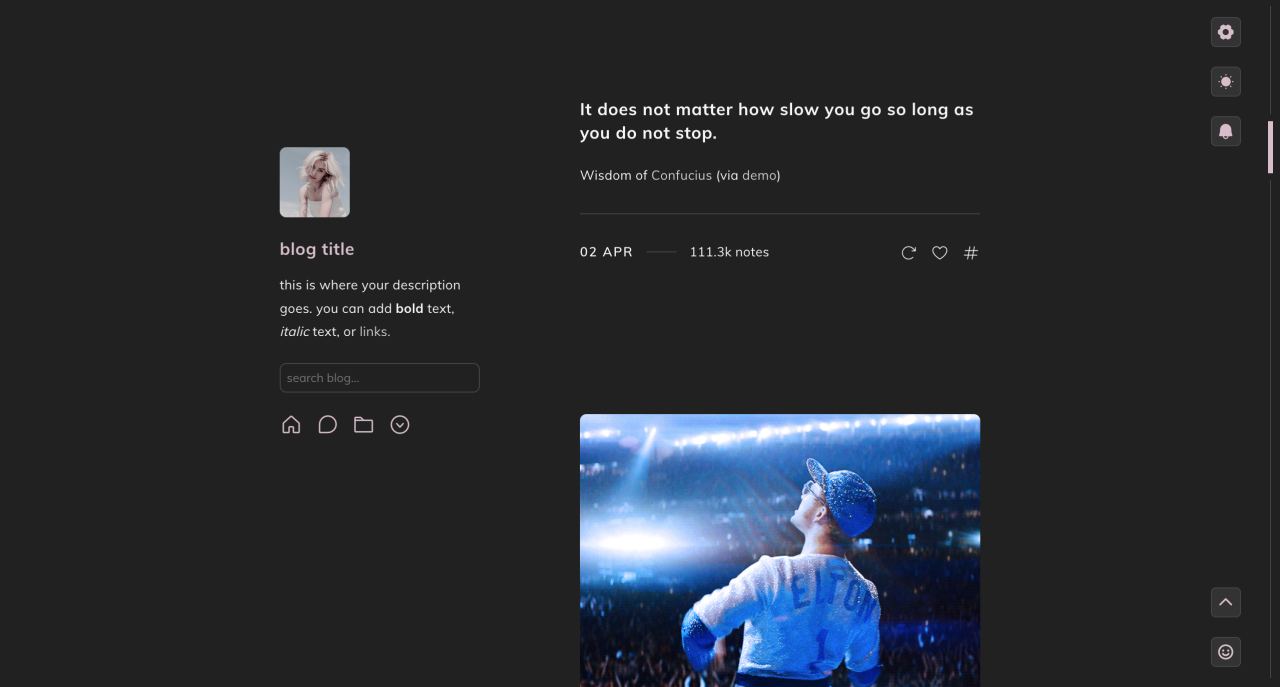### Blog Title
#### [Insert Blog Name] 

![Female with blonde hair](image-link)

**This is where your description goes. You can add bold text, italic text, or links.**

&nbsp;

Search Blog:  
[Search Bar]

---

#### Navigation Icons:
- **Home:** ![Home Icon](home-icon-link)
- **Speech Bubble:** ![Speech Bubble Icon](speech-bubble-icon-link)
- **File Outline:** ![File Icon](file-icon-link)
- **Dropdown Arrow:** ![Dropdown Arrow Icon](dropdown-arrow-icon-link)

&nbsp;

**Motivational Quote:**
> "It does not matter how slow you go, as long as you do not stop."  
> — Wisdom of Confucius via Demo

---

#### Post Details:
- **Date:** April 2nd
- **Notes:** 1.3K
- **Icons:**
  - ![Refresh Icon](refresh-icon-link)
  - ![Heart Icon](heart-icon-link)
  - ![Tag Icon](tag-icon-link)

---

### Event Description:
A person wearing a blue hat and glasses, with brownish or reddish hair, and a white short-sleeved shirt that says "Elton" in blue on the back, is performing in front of a crowd. They have blue sleeves underneath their white shirt. The performance is highlighted by bright lights and an enthusiastic audience.